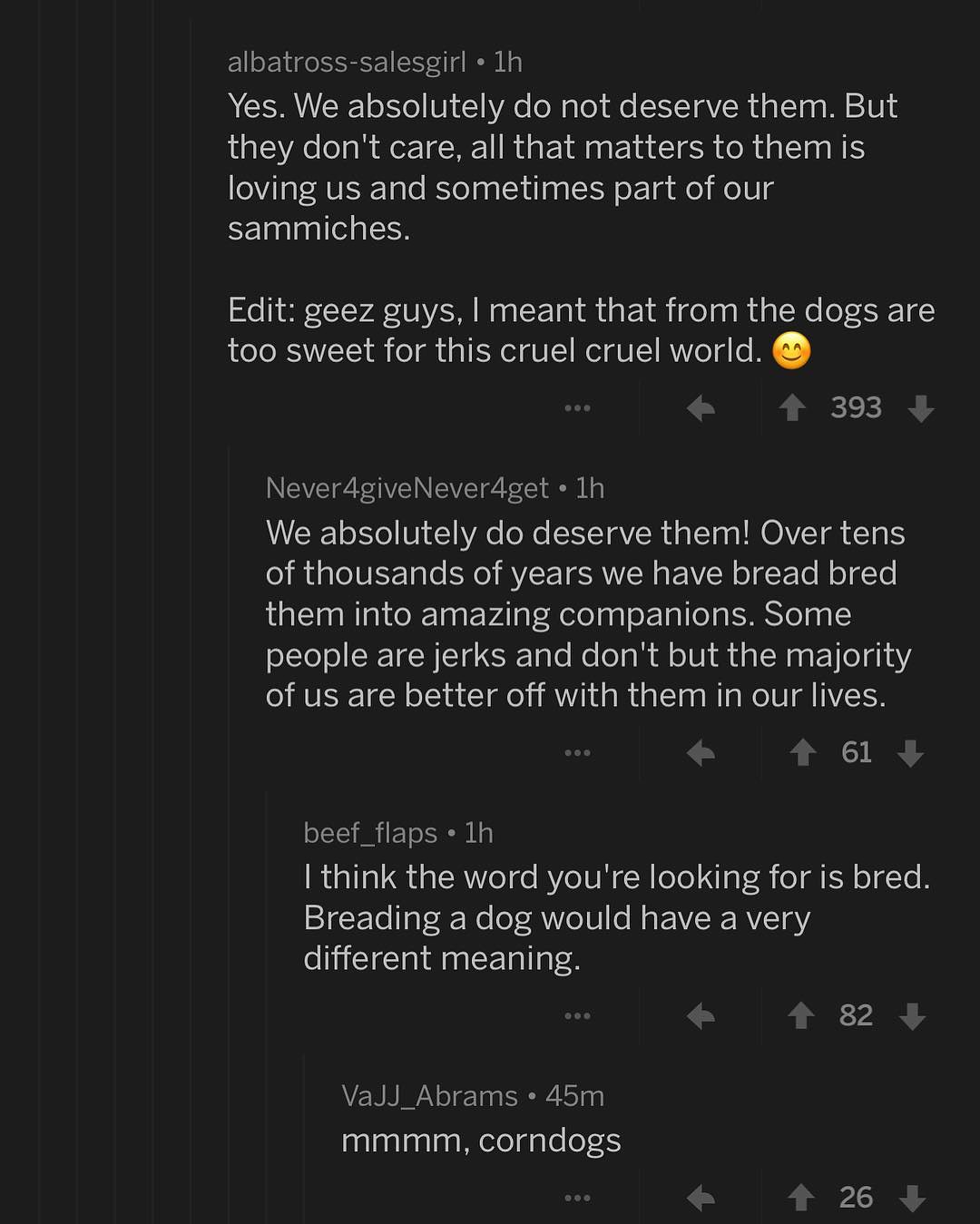The image is a screenshot of a chat from a social media platform displayed on a black background with white text. The conversation begins with a post by Albatross-Salesgirl, shared one hour ago, which reads: "Yes, we absolutely do not deserve them, but they don't care. All that matters to them is loving us and sometimes part of our sammiches. Edit: Geez guys, I meant that dogs are too sweet for this cruel, cruel world." This message received 393 upvotes. 

Following this, a user named NeverForgiveNeverForget commented one hour ago: "We absolutely do deserve them. Over tens of thousands of years, we have bred them into amazing companions. Some people are jerks and don’t, but the majority of us are better off with them in our lives," garnering 61 upvotes. 

Another user, Bflaps, also commented an hour ago, correcting the previous typo: "I think the word you’re looking for is bred. Breeding a dog would have a very different meaning," which got 82 upvotes. 

Lastly, 45 minutes ago, VAJJ_Abrams humorously replied with, "Mmm, corn dogs," receiving 26 upvotes. In the background, faint vertical lines, reminiscent of thin pen strokes, can be seen behind the text.